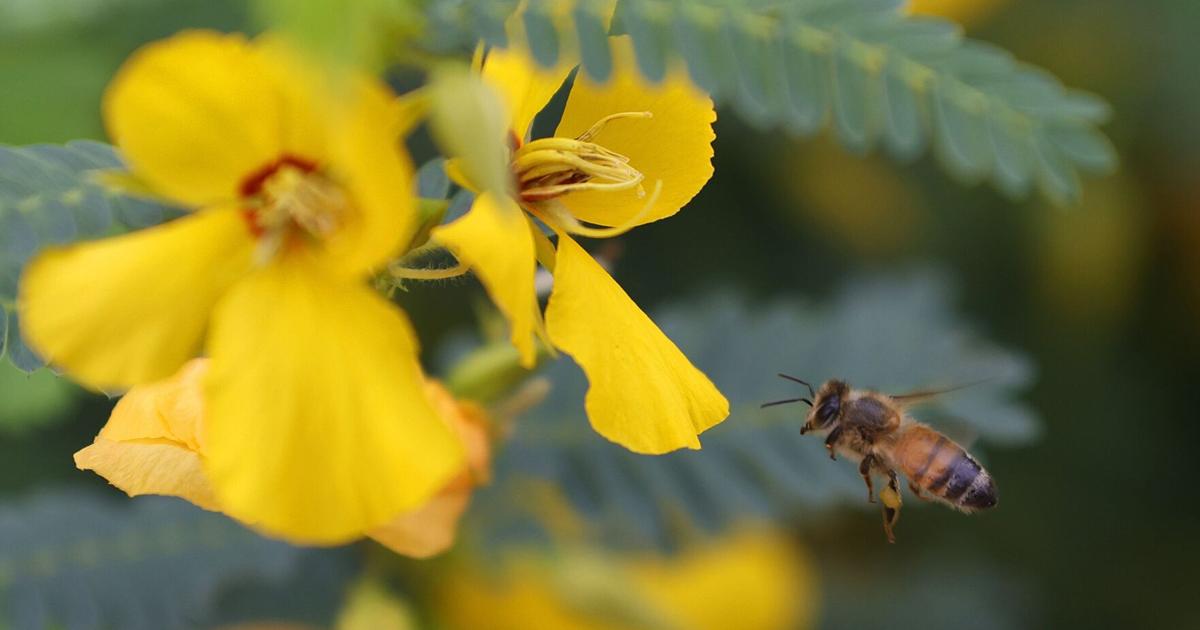In the photograph, a brownish-black honeybee with distinct black wings and antennas is captured in sharp focus as it flies toward a bright yellow flower with a red-edged pistil. The bee is mid-flight, preparing to pollinate the flower, which resembles a tulip or a lily, and stands out against a blurred background. There are two golden flowers, nestled on a green tree branch, with bluish-green leaves that frame the scene. The image, set in the daytime, employs a high depth of field to highlight the bee and a petal, making them the central focus amidst the softly blurred, shadowy surroundings.